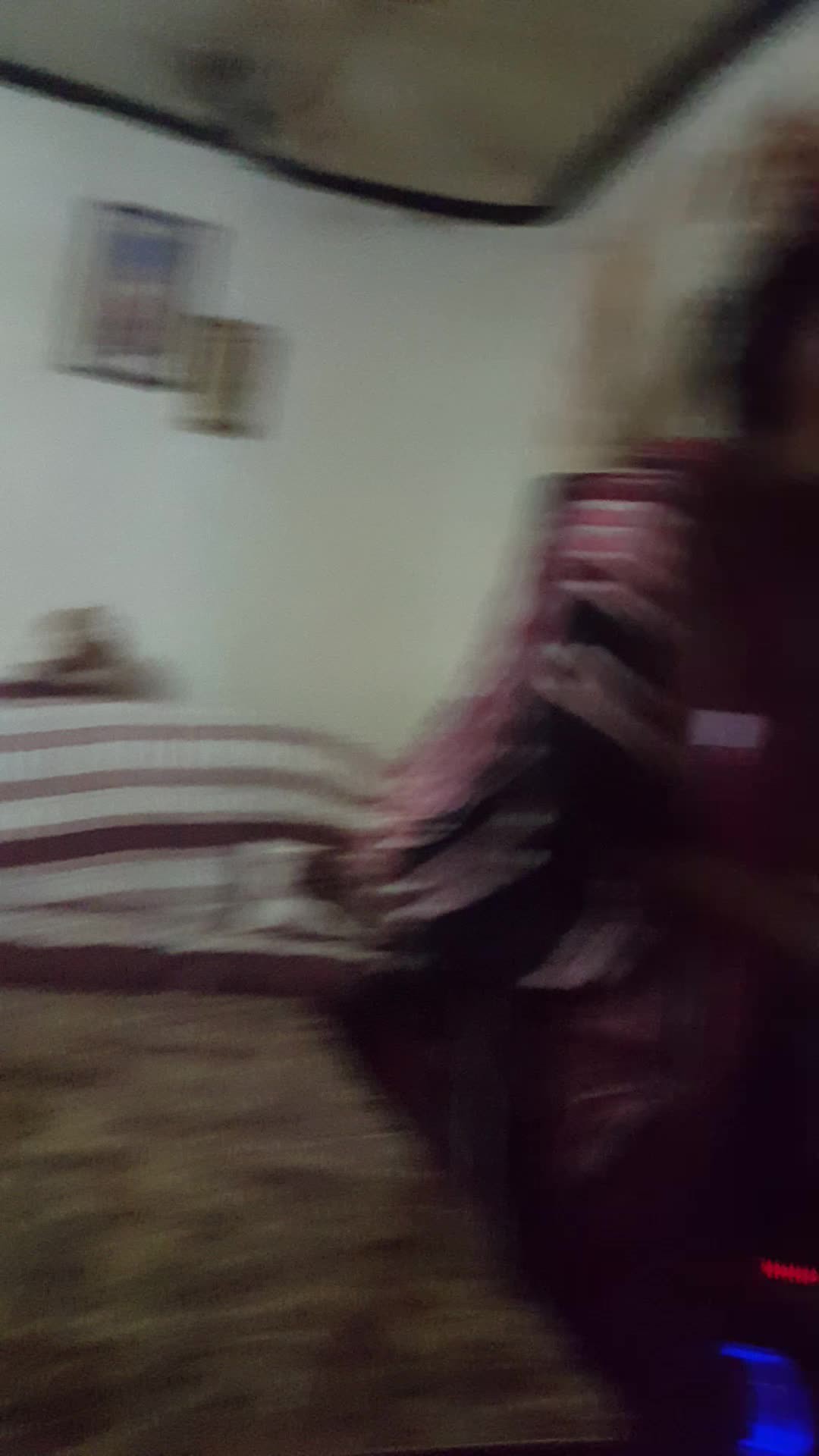The image is a very blurry photograph taken inside a room, making it hard to discern precise details. The room appears to have light-colored walls, possibly white, adorned with two framed pictures, one larger than the other. The walls meet a dirty-looking ceiling with brown or black trim, and the ceiling itself is also a brownish color. On the floor, which seems to be covered with tan or brown carpet, there are brown moldings along the perimeter of the room. A red striped object, which might be a blanket or some kind of fabric, extends across the view in a pattern that includes maroon and pinkish stripes, moving up and down. On the right side of the image, there's an ambiguous item that could be a console, piano, or perhaps even a bed, with a hint of blue in the bottom corner. The overall blurriness makes these details quite indistinct.